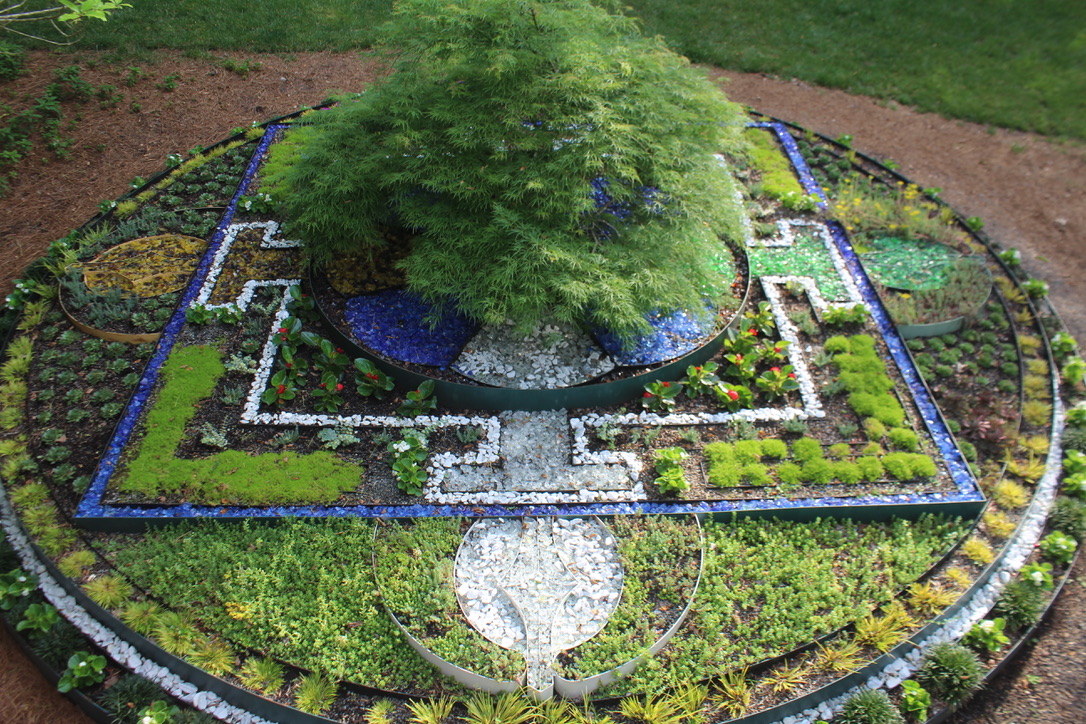The image captures an intricately designed, vertically rectangular garden bed viewed from above, with a striking central tree as its focal point. The garden is artistically divided into distinct sections forming a pattern reminiscent of a mosaic, with vibrant and contrasting colors. Around the central tree, there is a circle of white flowers bordered by green shrubs. Beyond this, a rectangular section with white flowers encloses green grass and red blossoms, with parts extending outward to create a dynamic shape.

Each part of the circular garden bed features varied plants—sections of blue, white, green, and brown hues forming distinct shapes. A path of small white stones weaves through the garden, enhancing the vivid colors of the vegetation. Surrounding the circular bed, patches of green grass and brown dirt frame the intricate layout. This beautifully landscaped garden, with its meticulous attention to detail and harmonious blend of colors and shapes, creates a visually captivating and serene outdoor space.